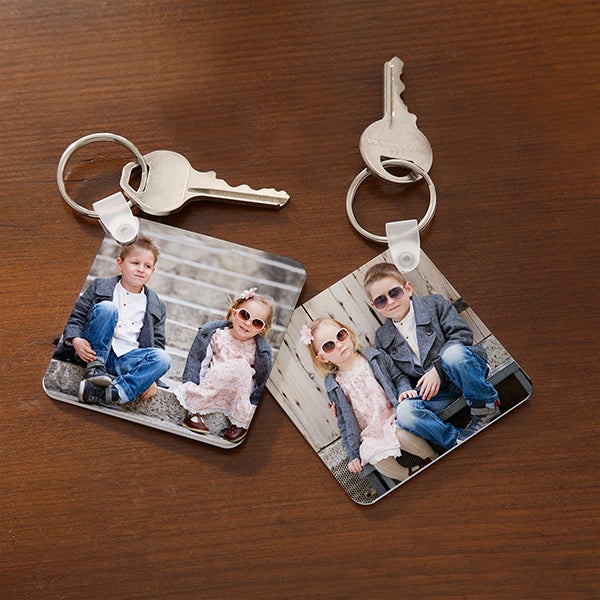This image showcases two silver metal keys laid on a dark wooden surface with a smooth grain. Each key is attached to a square keychain with rounded corners, displaying small photos. Both keychains feature the same young boy and girl, presumably siblings. In the photo on the right, both children are wearing sunglasses. The boy is dressed in a gray sports coat, white shirt, blue jeans, and tennis shoes, with one arm wrapped around the girl's shoulder. The girl is adorned in a pink dress, white tights, brown shoes, and a blue jean jacket, accented by a pink flower in her hair. They are seated closely together, exuding a sense of sibling affection. In the photo on the left, the children wear similar outfits, but the boy's sunglasses are either perched on his head or removed entirely. They are seated on concrete steps, with a small space between them. These charming keychains likely serve as personalized keepsakes for the owner, showcasing endearing images of their children.